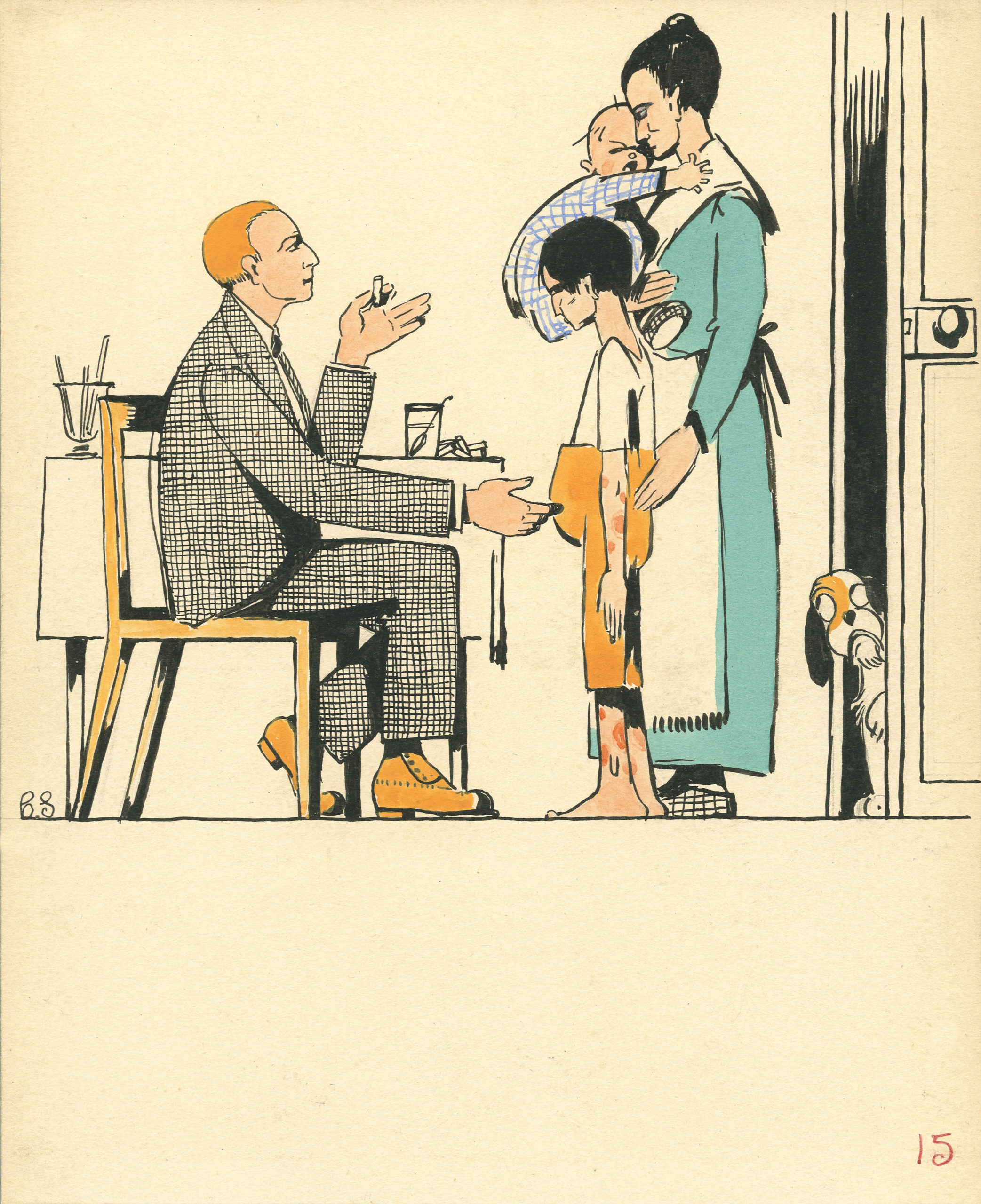The image is a detailed, colored pencil drawing set against a beige background, marked with the number 15 at the bottom and the initials "BS" on the left side. It features a man seated at a table on the left-hand side, dressed in a finely checkered black-and-white suit and brown button shoes. The man, who has reddish-blonde hair, is holding a cigarette in his right hand, which is extended upwards, while his left hand also holds a cigarette. In front of him stands a woman with black hair styled in a bun, appearing quite displeased. She is dressed in a seafoam green dress with a white apron, holding a crying baby in a blue-and-white outfit. Her left hand is placed on the lower back of a young boy with dark hair, who is looking down somberly. The boy is casually dressed in a white top and reddish-brown knickers that match the man’s hair and shoes. The child’s arms and visible parts of his legs are covered with red spots. To the right of the group, a partially open door reveals a dog watching the scene, seemingly frowning. On the table behind the man are a glass, some breadsticks, and other nondescript items.